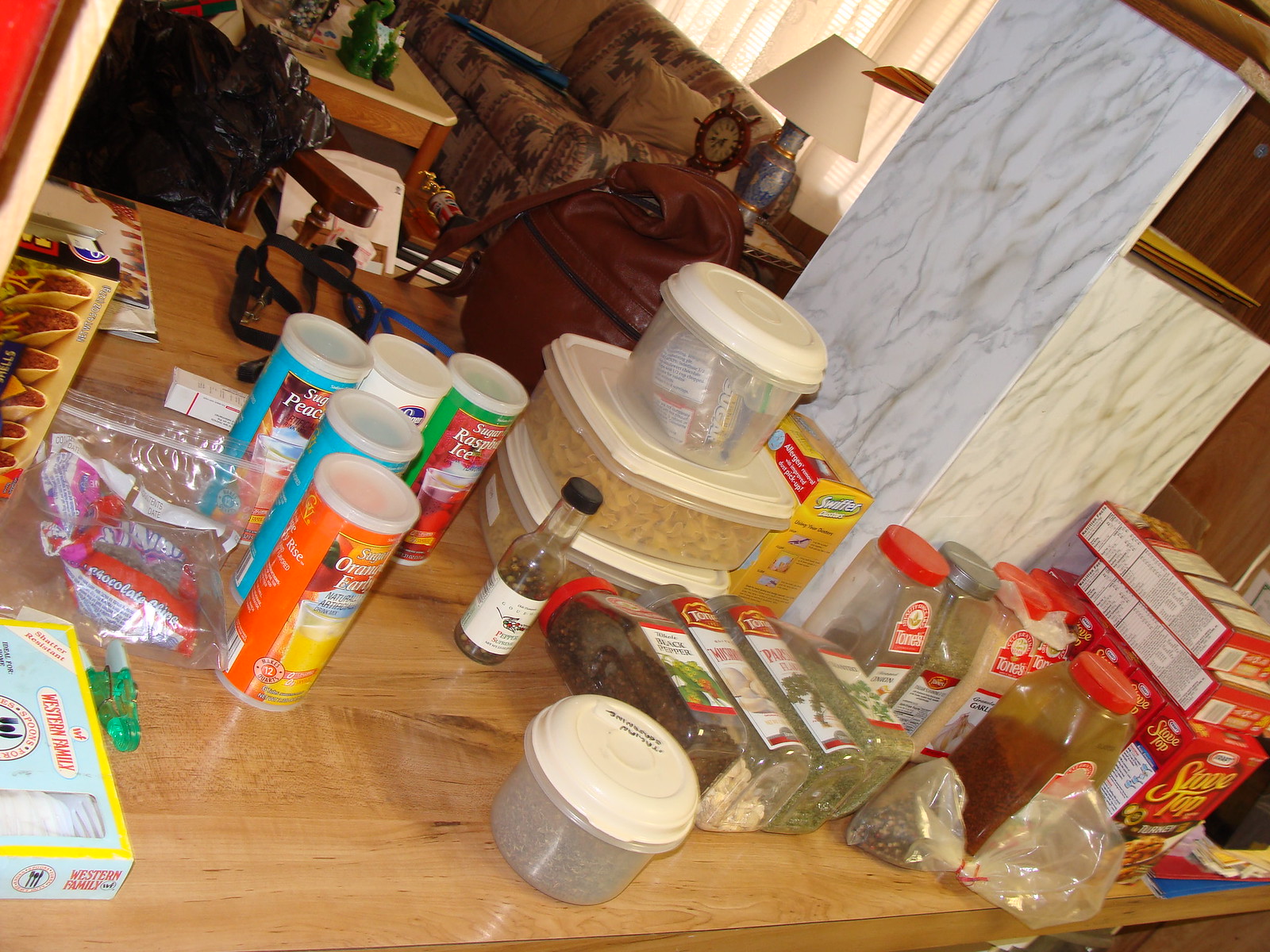The image showcases a bustling kitchen counter with a wood-like surface, cluttered with an assortment of items. On the far right, there are several boxes of stovetop stuffing. Next to them are large spice containers, and to their left, a bag is partially visible. Various spices are scattered across the countertop. Nestled among them are square and round Tupperware containers with white lids; one contains noodles. To the left of these containers, several iced teas or tea drink mixes are arranged in an L shape. Further left, a small baggie filled with candy can be seen. At the very bottom left, there is a container holding forks or other cutlery. The photo is taken at an unusual angle, providing a candid, slightly chaotic view of the space. Behind the stovetop stuffing boxes, a white marble-like box is partially visible. In the background, elements of a living room with furniture can be discerned, adding depth to the scene.